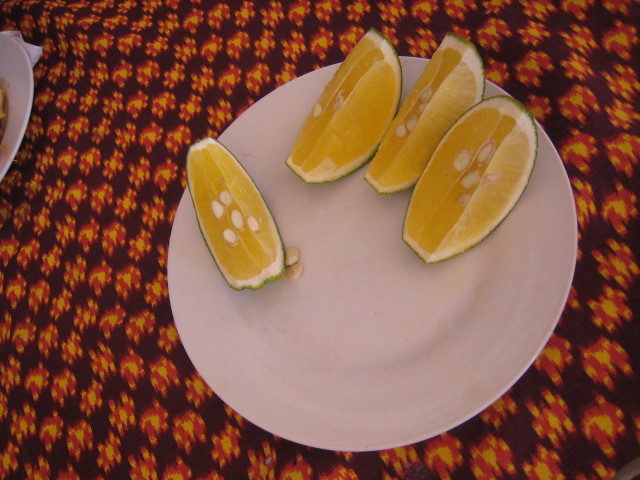The image features a vibrant tablecloth with a dark brown background adorned with an intricate pattern of circular shapes in shades of orange, yellow, and red, running vertically across it. Central to the photo, a white saucer holds a fruit cut into four segments. The fruit's orange flesh, abundant with seeds, contrasts sharply with its green rind, suggesting it could be an exotic citrus variety, reminiscent of an orange but with unique characteristics. One segment is positioned at the nine o'clock position with two seeds nestled beside it, while the remaining three segments are arranged from twelve to three o'clock, forming a semi-circle. Additionally, the table setting partially reveals another plate with indistinguishable contents off to the side. This carefully composed image, likely taken with a digital camera, captures the vivid colors and textural details of both the fruit and the decorative tablecloth, creating a rich, inviting scene.